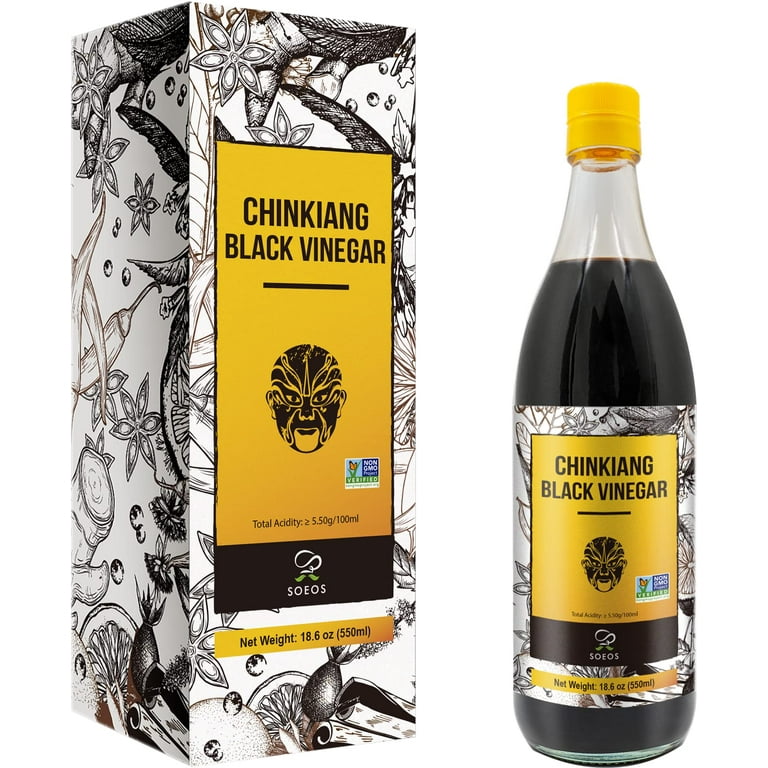The photo showcases a black vinegar product, highlighting both its packaging and the vinegar bottle. On the left side, there's a tall, thin, rectangular box with an ornate design. The box is primarily white with intricate black floral and citrus patterns, and possibly butterflies. A prominent gold label on the front reads "Chinkiang Black Vinegar" in black font, featuring a tribal mask as the logo. Below the logo, the label notes the total acidity (5.5 grams per 100 milliliters) and the net weight (18.5 ounces). The box also includes a non-GMO label and another label that says S-O-E-O-S.

On the right side of the photo is the vinegar bottle, which mirrors the box’s labeling with the same gold, black, and white ornate design. The bottle itself is glass, mostly full, and capped with a gold lid. The consistent design elements between the box and bottle create a coherent and striking visual identity for the Chinkiang Black Vinegar.